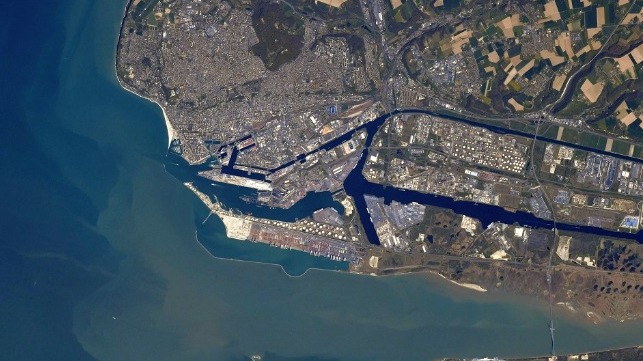An aerial photograph capturing a sprawling metropolitan city situated along a seashore. The cityscape, densely packed with buildings in shades of brown and beige, is punctuated by winding canals and a prominent river that sweeps from the upper left to the lower right, eventually merging into the sea. The river's entry forms a striking contrast of swirling brown against the deep blue of the ocean. High bluffs align the river, some too steep for construction but topped with homes. Industrial areas cluster near the waterfront, with notable structures like a jetty jutting into the sea. To the city's edge, farmlands stretch out, adding patches of green, while the bottom right reveals undeveloped areas rich with trees. This elevated view offers a comprehensive mosaic of the urban labyrinth, the vast expanse of water, and the contrasting natural landscapes.